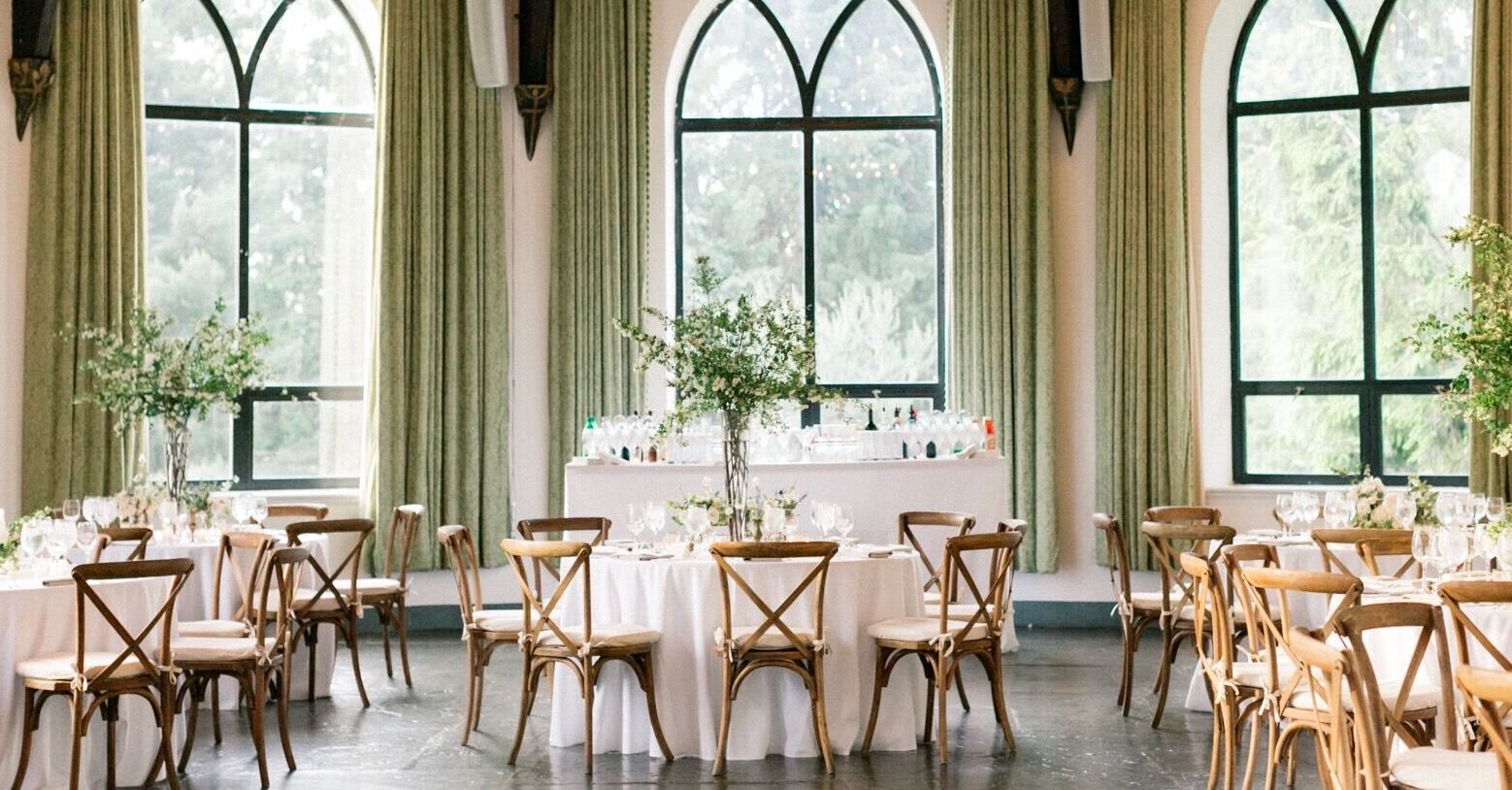This photograph captures the elegant setting of a dining room, possibly prepared for a wedding party. Dominating the scene are three large, evenly spaced arched windows that rise from the back wall, framed by rich green curtains that cascade from the ceiling. Each window showcases an intricate design resembling bullet outlines. Between these windows, thin pinkish strips of wall add subtle contrast to the vibrant decor.

In front of the central window, there's a prominent bar, adorned with an arrangement of glasses, hinting at a celebration. Surrounding this bar are several round tables, each draped with pristine white tablecloths. At the center of each table, vases filled with white roses or flowers, possibly accompanied by smaller vases, enhance the sophisticated atmosphere. Chairs, made of wood with white cushions, encircle these tables, ready for guests.

The overall layout features at least four such tables arranged symmetrically, with two on the left and two on the right side of the shot. A vase with a green plant adorns the center of each table alongside some silverware. The grayish floor completes the understated elegance, tying together the room's festive and refined ambiance.